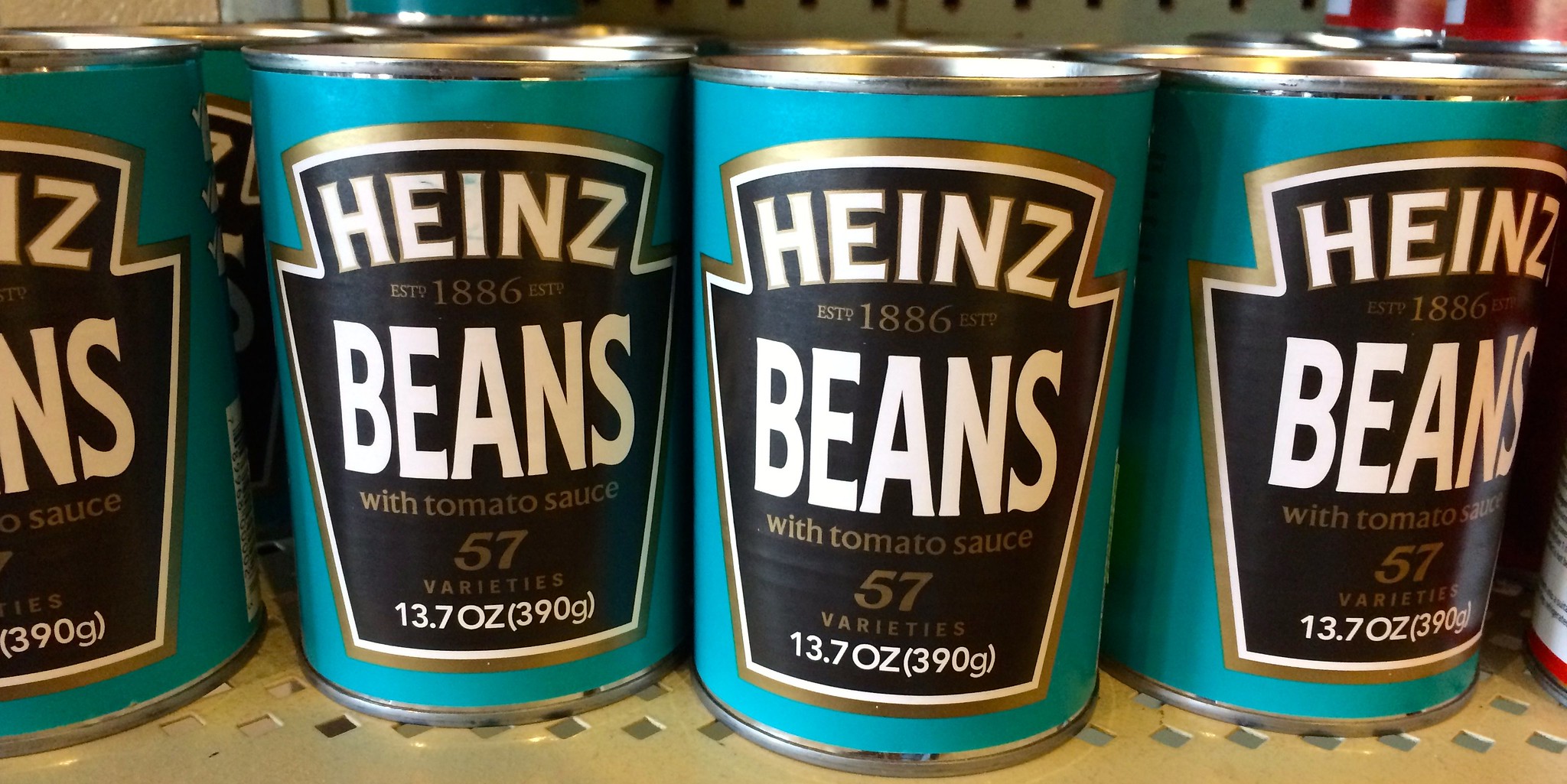The image depicts four Heinz beans cans on a metal shelf with a lattice design cut into it. The cans are primarily silver with bright turquoise blue labels, each bordered in gold. The labels prominently feature the Heinz brand name in large white lettering, along with "Beans" in equally large white letters. Below, in smaller white text on a black background, are the details: "Established 1886," "with tomato sauce," "57 varieties," and "13.7 ounces (390 grams)." The cans are well lit, making the reflective surface slightly shiny. The image is in landscape orientation, showing three full cans, half of another, and a sliver of yet another can on the side.